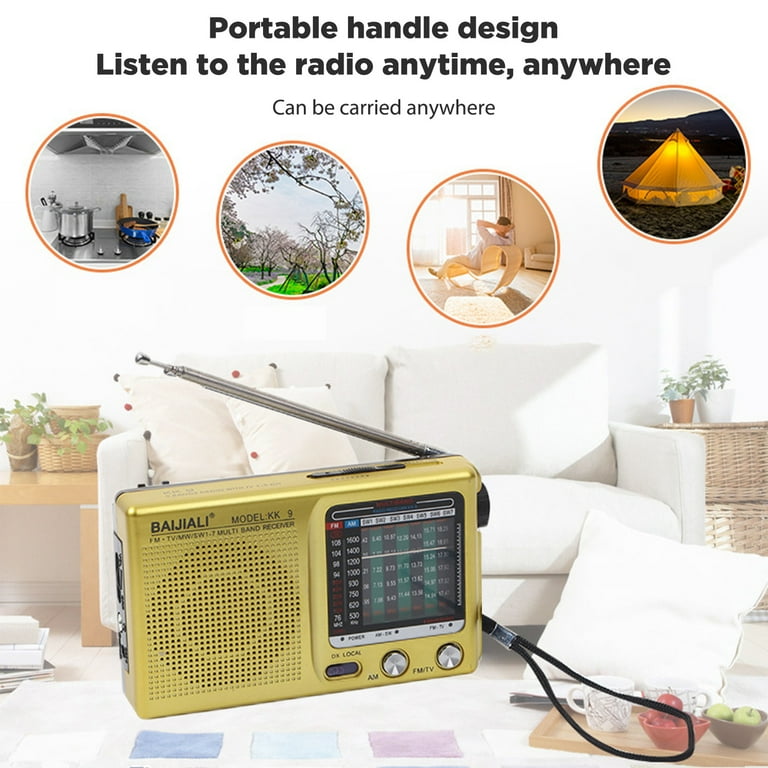The image is a product photo of a vintage-style, triangle-shaped yellow radio with a portable handle design, perfect for listening to the radio anytime, anywhere. The text at the top center, bold in black, reads, "Portable handle design, listen to the radio anytime, anywhere," with smaller text underneath, "can be carried anywhere." The radio features an extendable antenna, currently retracted, a lanyard for easy carrying, and a speaker with a dotted pattern on the left front side. Its right side showcases a large dial with lines indicating different radio bands, marked in green and black columns with white numbers, alongside an AM and FM button at the bottom. Branded as Bajiali, model KK9, the radio is placed against a white love couch background with wicker baskets and small potted plants, suggesting a cozy living room setting, albeit digitally enhanced.

Below the main text are four circular insets illustrating versatile usage scenarios: a kitchen stove with pots, a scenic outdoor path lined with trees, a person lounging in a modern indoor chair with sunlight streaming through the window, and a yurt-style tent outdoors. These images emphasize the radio's portability and suitability for various environments, from indoor leisure to outdoor adventures. The intricate settings and detailed product features suggest a listing image typical for online marketplaces like Amazon.